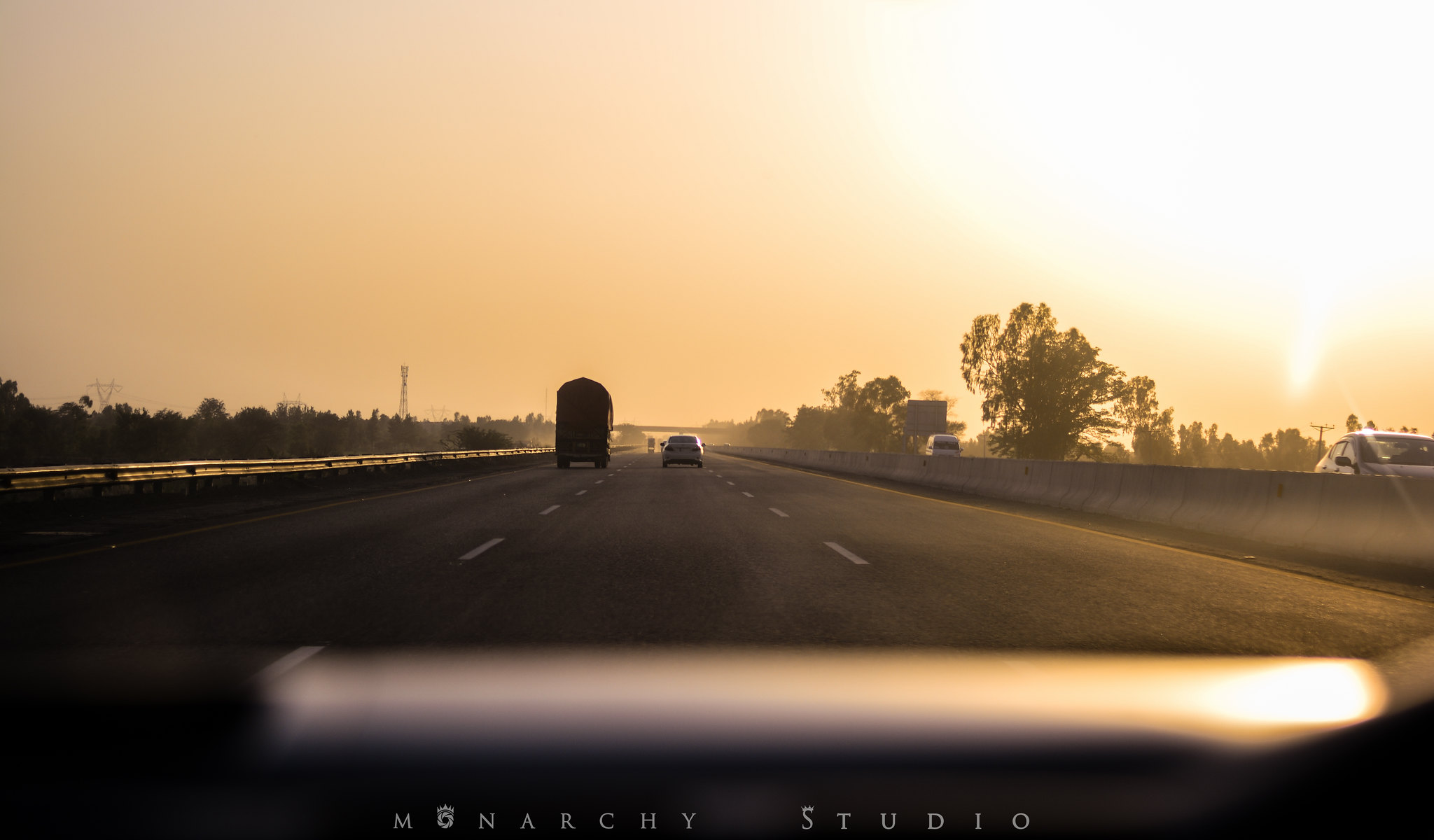The image captures a photograph from the center lane of a three-lane highway, taken from the perspective of a vehicle’s windshield. In the center lane, directly ahead of the vehicle, there is a small car, and in the far right lane, a large truck or tall bus is visible. To the right edge of the image is a concrete barrier that separates the oncoming traffic. Beyond this barrier, two cars are traveling in the opposite direction. The left and right sides of the road are flanked by trees, adding a touch of natural scenery. The sky displays a vivid pinkish-red hue, suggesting that it is either dusk or dawn, with the sun glowing faintly from the upper right part of the image. In the far distance, an overpass and what appears to be a cell phone tower can be seen. Across the bottom of the photo is a watermark that reads "Monarchy Studio."